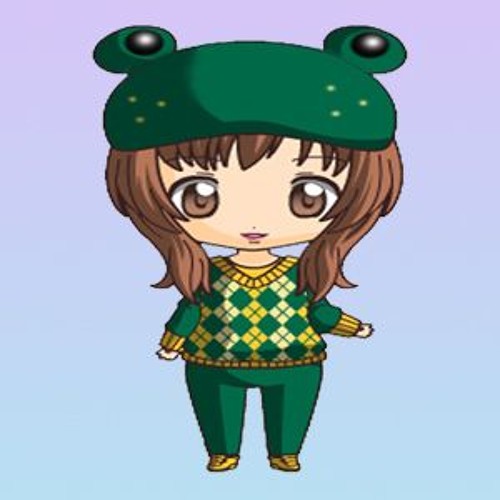In the cartoon image, a whimsical character takes center stage, her design exuding an exaggerated charm. Her head is notably larger than her petite body, creating a playful, disproportionate aesthetic. Her almond-shaped face is framed by rich brown hair that cascades past her shoulders, complemented by matching brown bangs. Perched atop her head is a quirky green hat designed to resemble a frog, complete with frog eyes sitting at the crown like whimsical ears.

The character is dressed in green pants and vibrant yellow shoes. Her upper attire is a unique sweater, where the sleeves are green with yellow cuffs, creating a harmonious blend with the green and yellow diamond pattern adorning the rest of the sweater. Her facial expression is one of curiosity or excitement, with her mouth slightly ajar, revealing a hint of personality.

Her eyes are strikingly large, predominantly white with a brown iris that encloses a smaller white circle, giving her a look of perpetual wonder. The background against which she stands features a soothing ombre gradient, transitioning from deep purple at the top to a lighter periwinkle hue towards the bottom, adding a dynamic and dreamy quality to the overall scene.